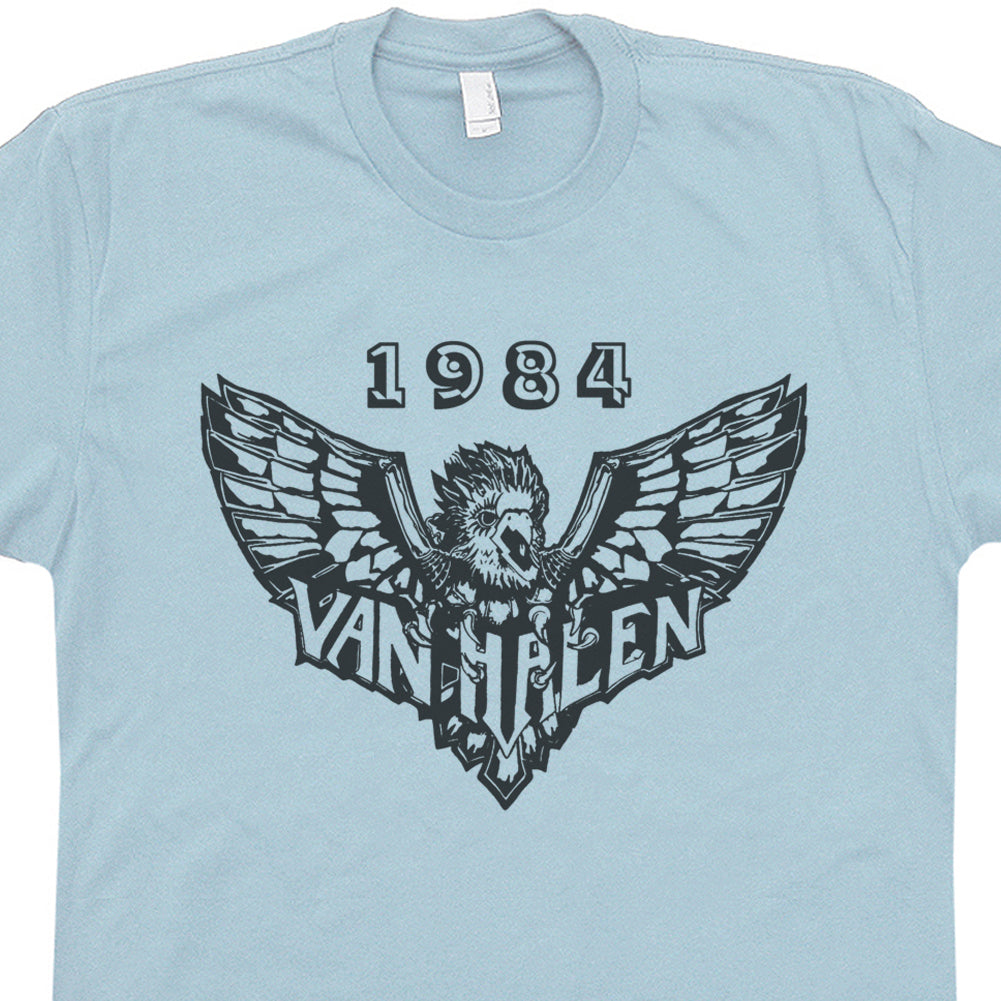The image showcases a light pale blue Van Halen band t-shirt, positioned against a plain black background. The t-shirt, likely vintage, features a rounded collar with a visible but unreadable size tag at the back. Dominating the center of the shirt, in bold black lettering, is the year "1984." Beneath these numbers, a dynamic design of a predatory bird, likely an eagle or hawk, is depicted with outspread wings and fierce expression. The bird's powerful talons grasp and seem to rip through the letters forming the band's name, "Van Halen," which is also outlined in black. Despite being a simple and stark image, the detailed representation of the bird and the band’s name create a striking, bold graphic on the shirt.